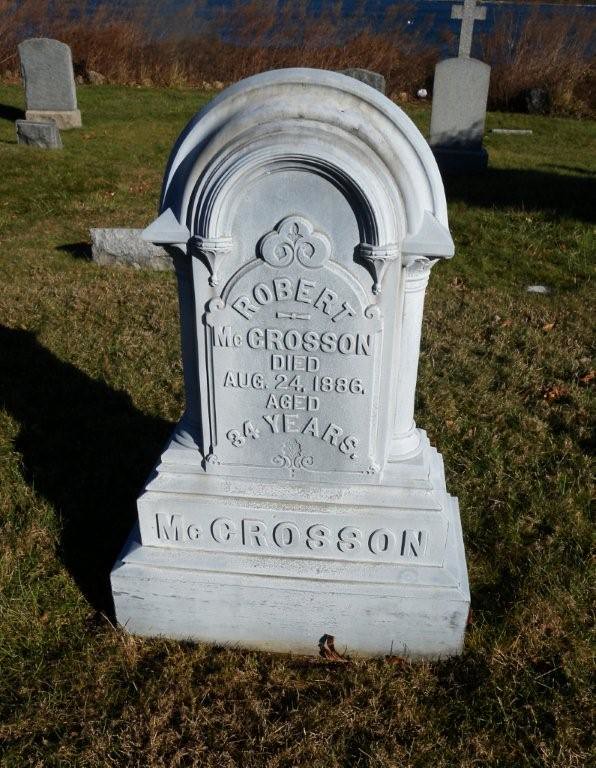The photograph depicts a cemetery scene centered around a prominent white tombstone made of stone, inscribed with the text: "Robert Macrossone, died August 24, 1886, aged 34 years," with "Macrossone" prominently displayed at the base. The tombstone features a curved top and sits atop a substantial base. The setting shows a mix of green and brown grass in both the foreground and background, indicating a possibly dry season, likely fall or winter. Surrounding the main tombstone are several other gravestones, including a shorter rectangular one immediately behind, a square-shaped one to the left, and others with various shapes including one with a cross on top. The background features overgrown orange and brownish weeds or dead trees, adding to the scene's somber and aged atmosphere. The well-manicured grass in the foreground contrasts with the more wild and overgrown state of the vegetation in the background. The scene is clearly captured in daylight, with shadows cast by the tombstones enhancing the depth of the image.